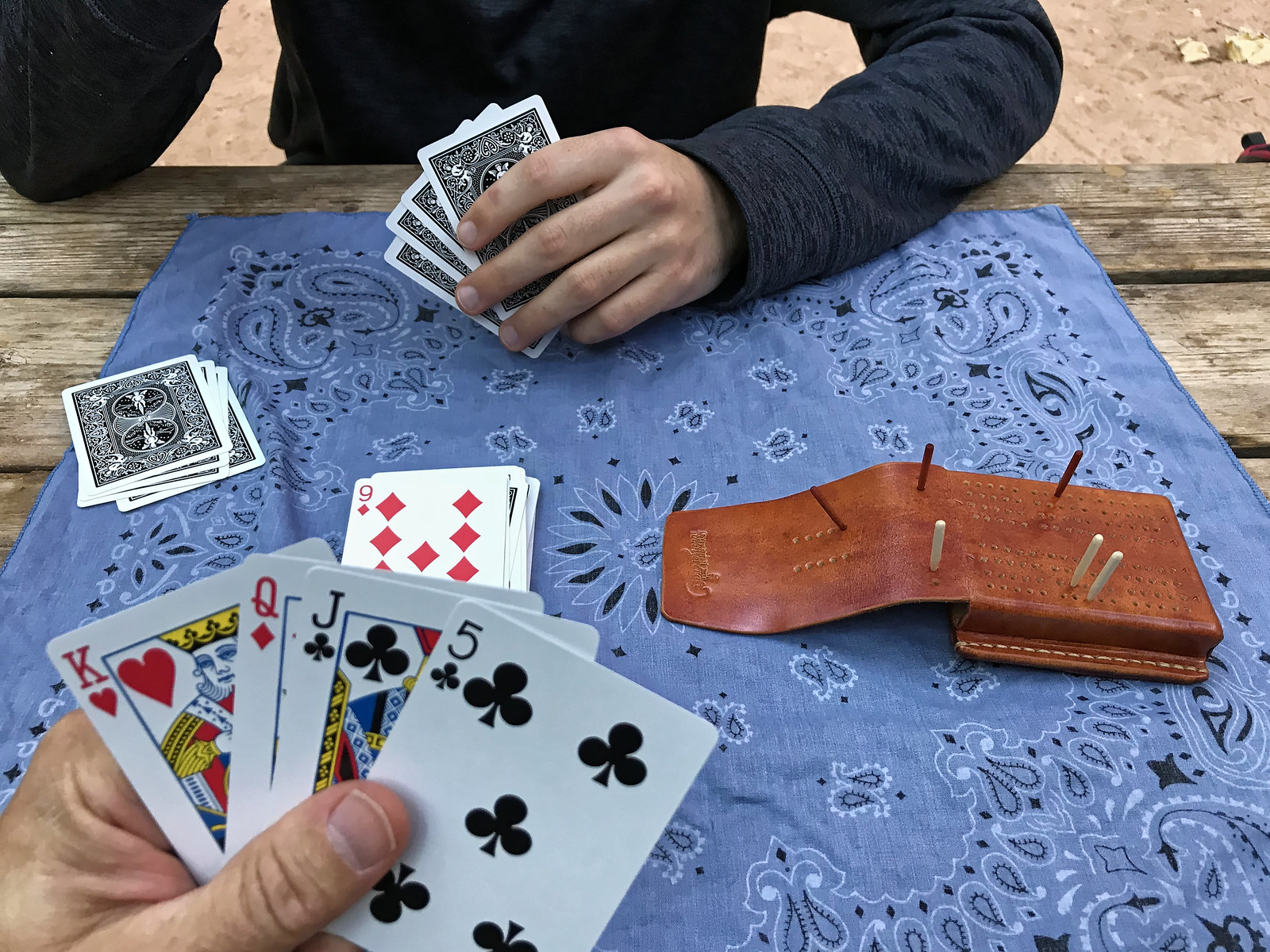In this evocative photograph, two individuals are deeply engaged in a game of cards. The image is captured from the perspective of one of the players, focusing on their opponent who sits across a weathered gray wooden table reminiscent of a picnic setup. The background reveals exposed brown earth, adding a rustic ambiance to the scene. 

In the foreground, the partial view of the player's hand displays a set of four cards: a King of Hearts, Queen of Diamonds, Jack of Clubs, and Five of Clubs. The player’s pale-skinned hand emerges from the lower left corner, subtly anchoring the viewer’s perspective. 

Their opponent, visible on the opposite side of the table, has fair skin and is dressed in a long-sleeve dark gray shirt. The opponent's concentration is palpable as they contemplate their next move, their hands and part of their upper body illuminated in the soft light.

The playing surface is a blue patterned handkerchief laid out carefully on the table, adding a splash of color and texture. On the left side of the handkerchief, a small stack of four face-down cards lies in a slightly uneven pile. In the center, a taller stack of cards with a nine of diamonds face up on top suggests the dynamics of the game in progress.

Adding intrigue to the scene is a brown leather object on the right, resembling a wallet. This object is punctuated with small holes and contains wooden pegs, six in total—three white and three red—carefully inserted into these holes. The arrangement hints at a scoring system or an additional game connected to the card play, enriching the layers of engagement between the participants.